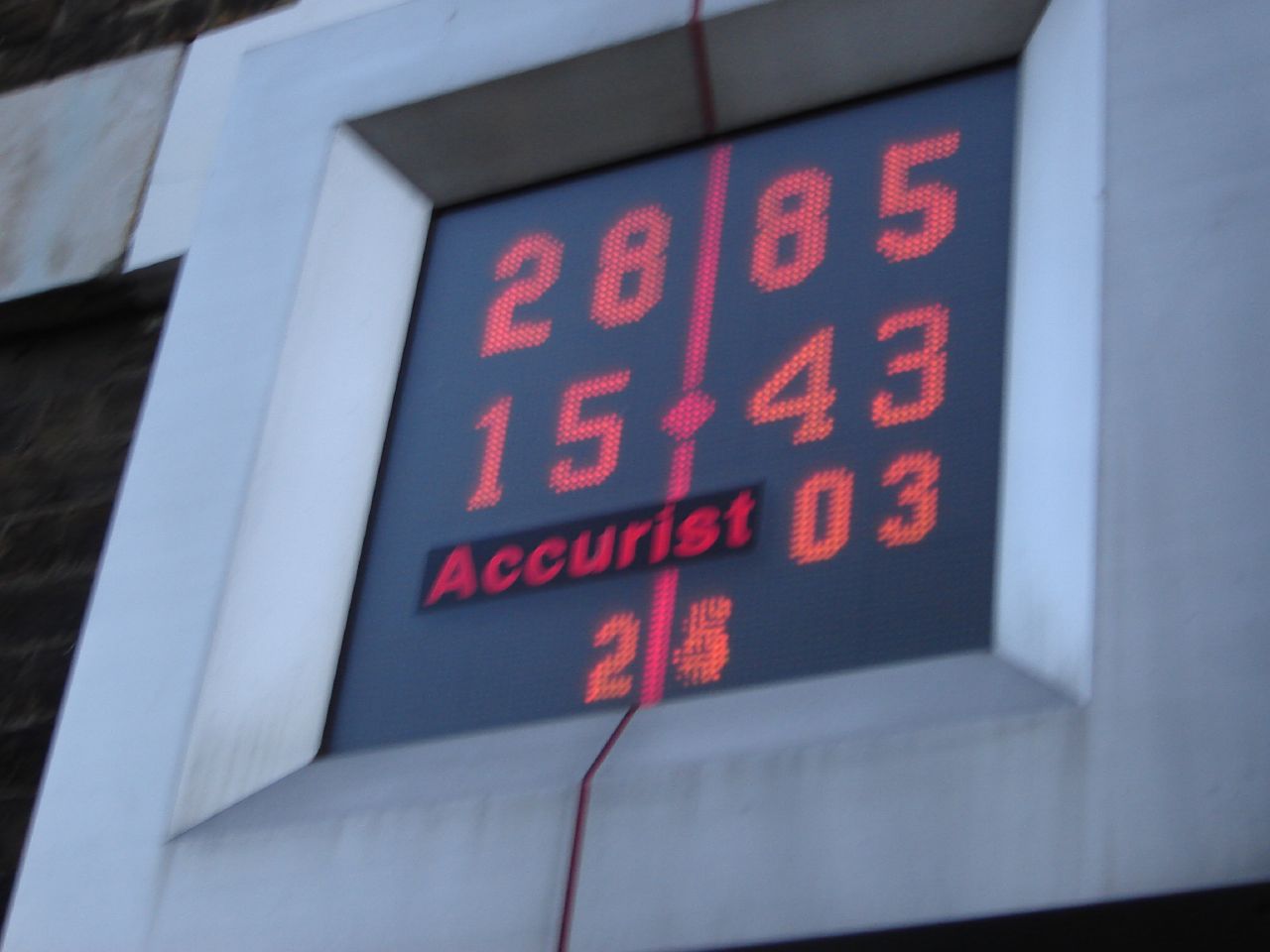The photograph depicts an out-of-focus digital display housed within a robust stone or concrete frame, characterized by bevels at the corners and a vertical seam tinted red running through its center. The seam bisects the frame and the corresponding digital screen inside, which is black and features a scattering of red numbers. At the intersection of the seam is a diamond shape. The displayed numbers from left to right read 2, 8, 8, 5, 1, 5, 4, 3, 0, 3, followed by an indistinct blur. To the left of the "03," the word "Accurist" appears in red letters below the "15." The stone frame gives the image a heavy, substantial appearance, while the white-grayish backdrop of the wall further contrasts with the dark screen and vibrant red details.